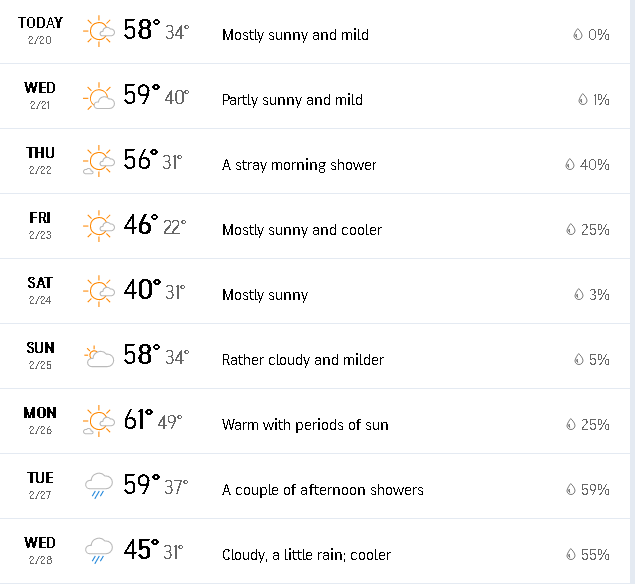The image displays a detailed weekly weather forecast as follows:

- **Tuesday, 2/20**: Mostly sunny and mild with a high of 58°F and a low of 34°F. Minimal cloud cover, 0% chance of precipitation.
- **Wednesday, 2/21**: Partially sunny and mild with a high of 59°F and a low of 40°F. Slight cloud presence with a 1% chance of rain.
- **Thursday, 2/22**: Sunny with intermittent clouds. High of 56°F and a low of 31°F, with a 40% chance of a stray morning shower.
- **Friday, 2/23**: Mostly sunny and cooler, with a high of 46°F and a low of 22°F. Partial cloud cover and a 25% chance of precipitation.
- **Saturday, 2/24**: Mostly sunny with a high of 40°F and a low of 31°F. Slight cloud presence and a 3% chance of precipitation.
- **Sunday, 2/25**: Rather cloudy and milder with a high of 58°F and a low of 34°F. Partially cloudy with a 5% chance of precipitation.
- **Monday, 2/26**: Warm with periods of sun. High of 61°F and a low of 49°F. Mostly sunny with a 25% chance of precipitation.
- **Tuesday, 2/27**: Expect a couple of afternoon showers with a high of 59°F and a low of 37°F. Overcast conditions with a 59% chance of precipitation.
- **Wednesday, 2/28**: Cloudy with a little rain and cooler temperatures. High of 45°F and a low of 31°F. A 55% chance of precipitation.